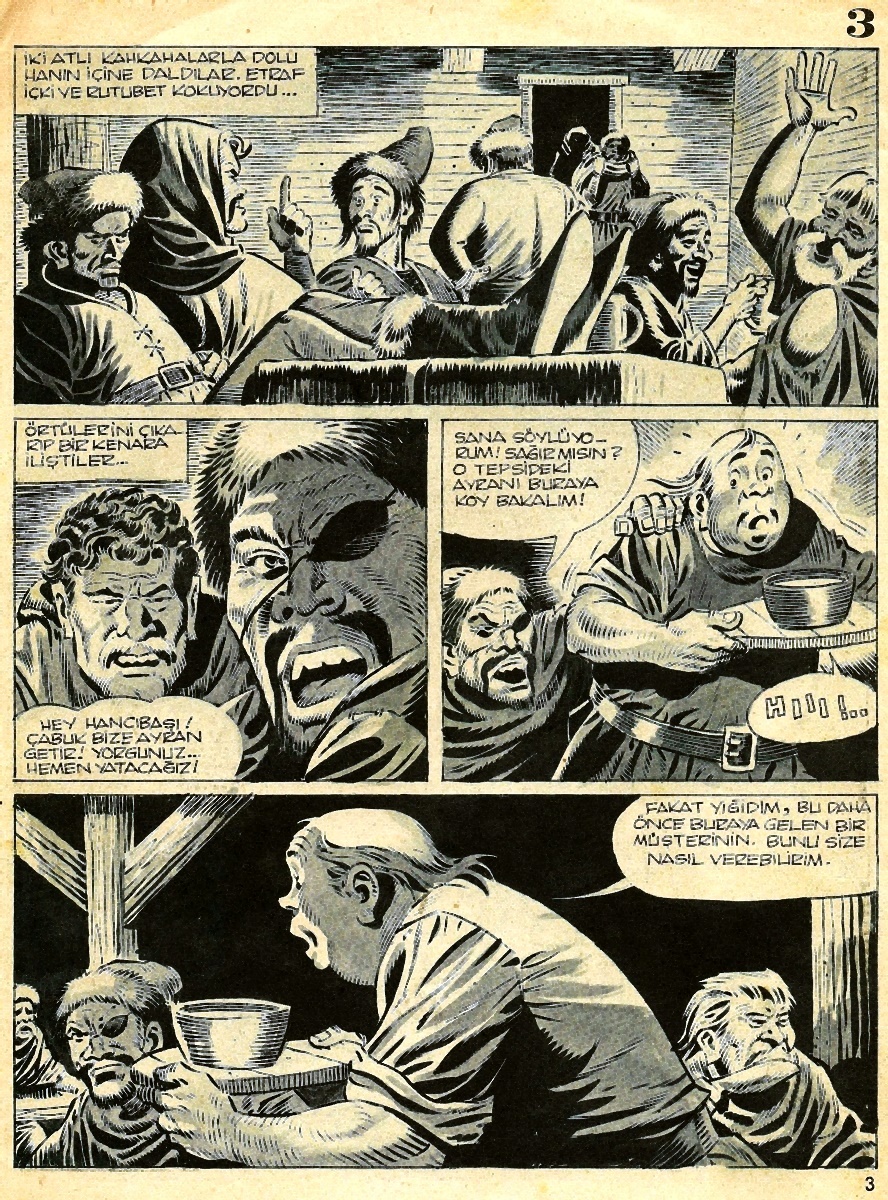This image is a black-and-white cartoon page from an antique newspaper or graphic novel, featuring three detailed strips, set in a foreign language possibly Mongolian or Turkish. The page is yellowed with age, and a faint white border is visible at the top. There is a number three in the upper right corner, indicating the page number. Each strip illustrates scenes with characters dressed in medieval-style clothing such as robes and togas.

In the first strip, a group of men is depicted sitting around a large wooden block or table, engaged in conversation. One man has his hand raised while another, with his feet on the table, joins the discussion.

The second strip is divided into two parts. The left half shows a man with an eyepatch, mouth open, seemingly yelling in an unknown language, with another man seated beside him. The right half portrays a server carrying a bowl on a tray, being touched by another figure.

The final strip continues the interaction in what looks like an alehouse. It shows the server with the bowl talking to the man with the eyepatch, as another man stands behind them.

Overall, the detailed illustrations and the setting suggest a historical or nomadic theme, capturing an intense scene, likely in a communal or dining environment.